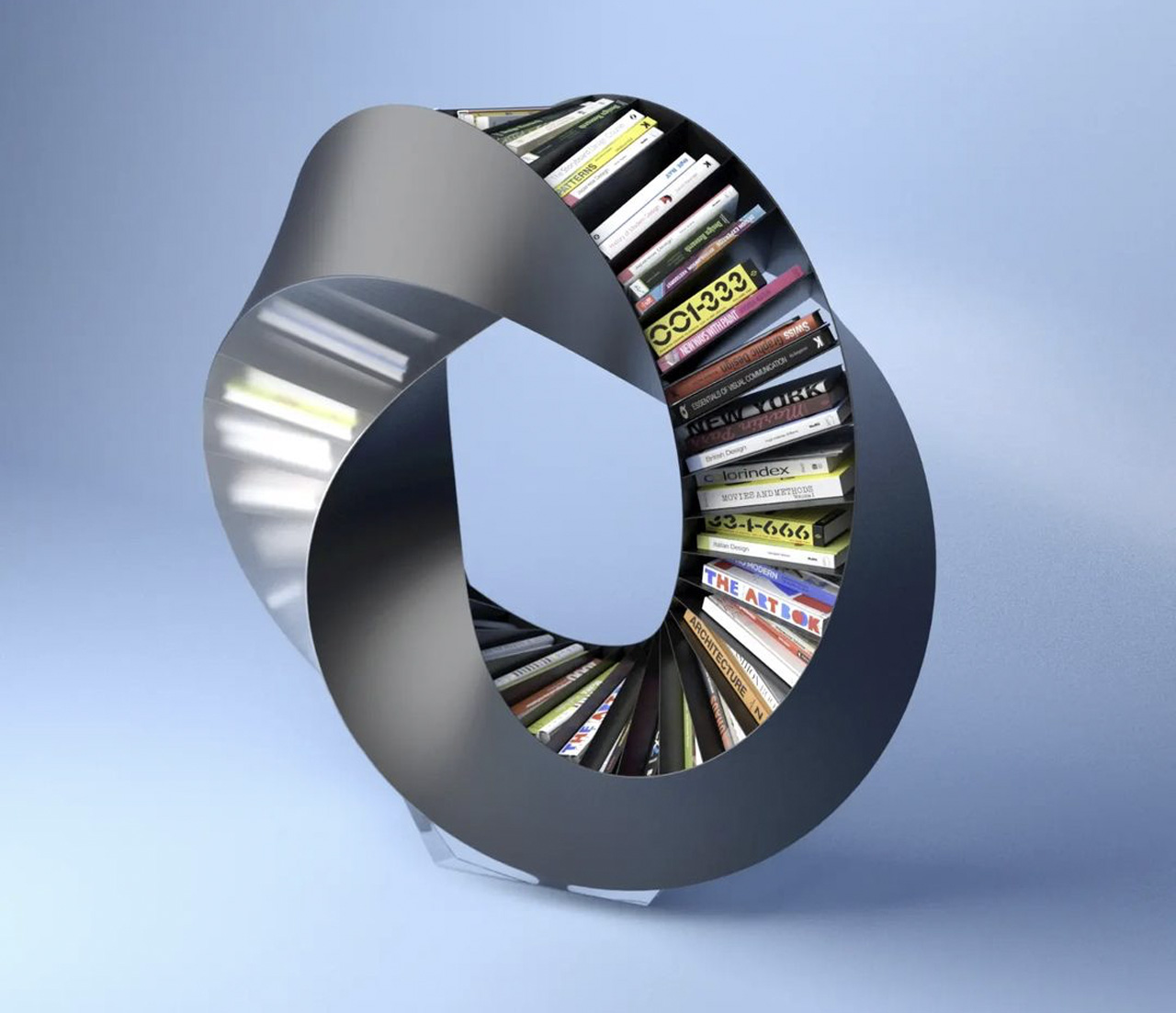This image features an abstractly shaped, surreal bookshelf with a sculptural design that spirals and twists like an intricate knot or pretzel. Made of metal, the bookshelf has a striking silver or gray color with transparent elements on one side and some open slots on the other. The spiral structure supports various books that are arranged irregularly, some appearing to defy gravity. Notably, the spines of two books or cassette tapes display the numbers "001-333" and "3-1-666," while the other titles remain illegible. The artwork, backed by a powder blue background with soft shadows in the top left and bottom right corners, evokes a sense of movement and fluidity, enhanced by bars of white light on one side of the structure.